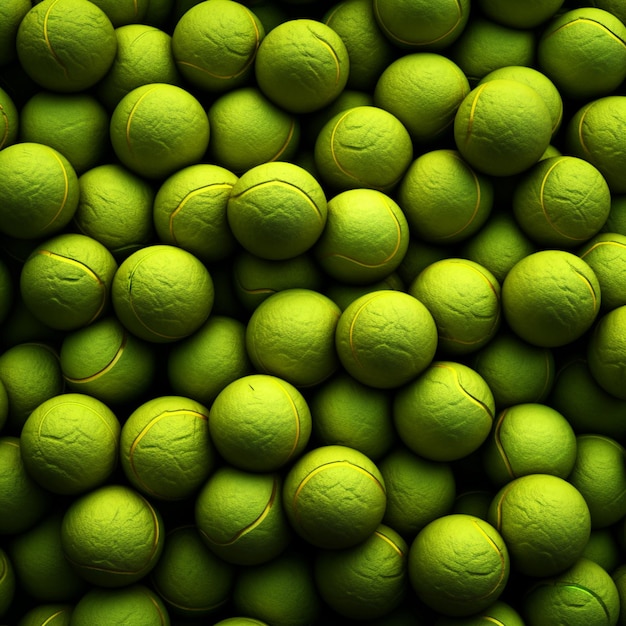The image depicts a tightly packed pile of lime green balls, each about the size of a tennis ball, with numerous of them stacked on top of each other. The balls feature a lighter green, narrow ridge or seam similar to the white lines seen on tennis balls, but the lines are incomplete, and the surface is noticeably textured and wrinkled, unlike the typical smooth surface of a standard tennis ball. These balls might resemble tennis balls at a glance, but their irregular surface suggests they could be something else entirely, such as a type of fruit. The shadowing between the balls creates dark gaps, causing parts of the pile to appear almost black. Overall, the dense arrangement and uniformity of the balls create a visually intriguing and somewhat ambiguous scene.